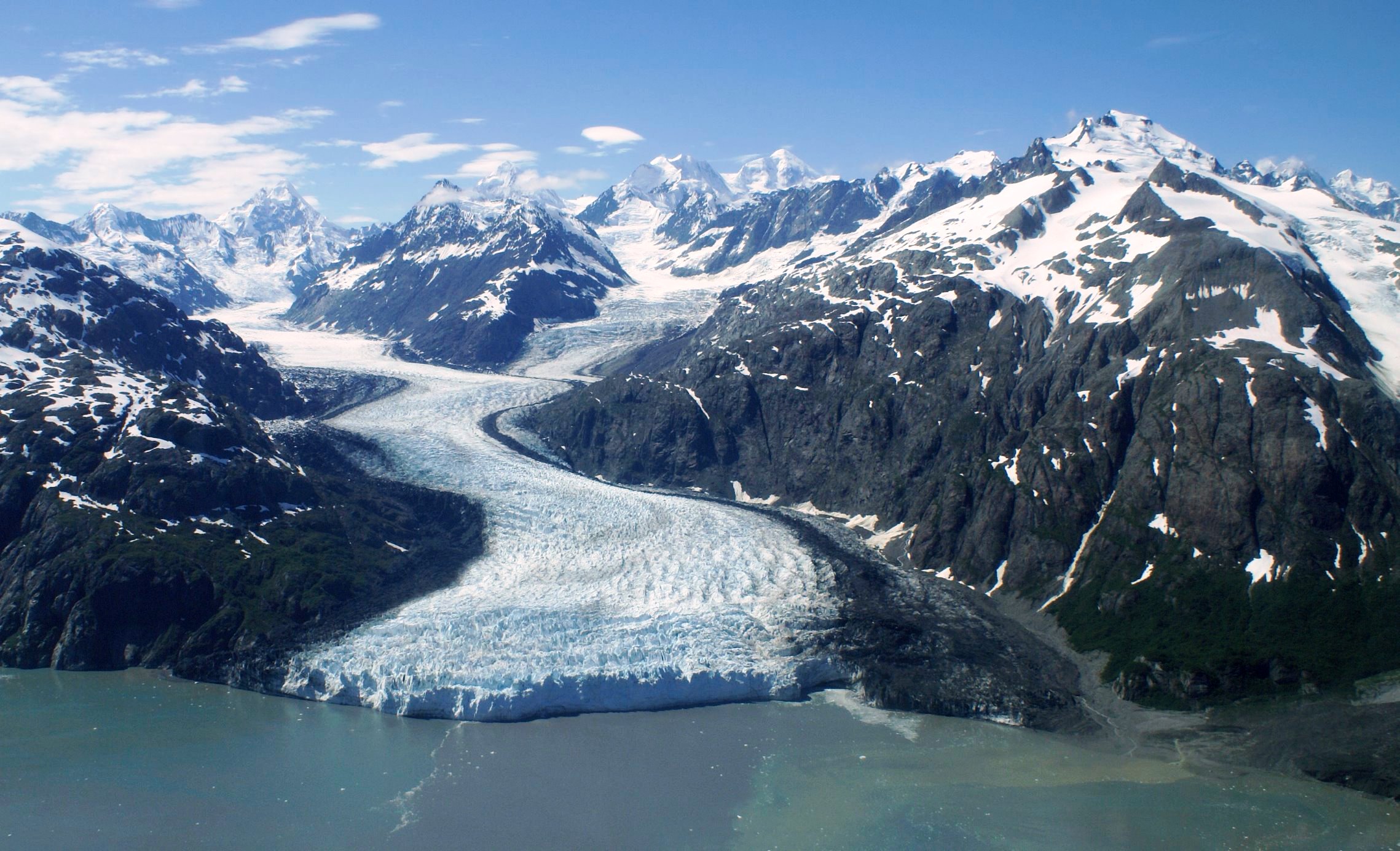This stunning aerial photograph showcases a breathtaking glacial landscape. Dominating the center of the image is a wide, winding river of ice leading down into an expansive ocean or lake in the foreground. The ice pathway is thick, snow-covered, and distinctly flanked by towering black mountain ranges. The peaks of these mountains are dusted with snow, while their faces are primarily black with specks of white. These mountain ranges stretch out majestically, their rugged terrain interspersed with patches of moss or grass near the bases. The sky above is a serene blue, punctuated by a few wispy clouds predominantly to the left side, adding to the overall scenic beauty of this remote icy wilderness.